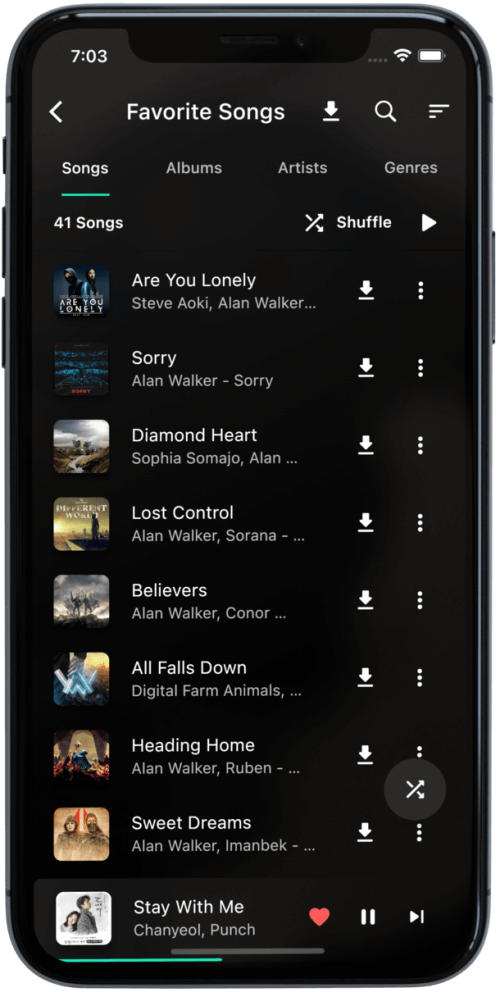The screenshot captures the display of a music application on a tablet. The tablet has a black border encasing the screen, which features a dark gray background. The top of the screen shows the current time "7:03" alongside a full battery icon. Below these indicators, an arrow points to the left, preceding the bold, large white text "Favorite Songs". There is also a download icon and a magnifying glass icon adjacent to the large text. 

Further down, the interface lists categories such as "Songs", "Albums", "Artists", and "Genres", with "Songs" highlighted by an underlined green line. The display indicates there are "41 songs" in the selected category. Each song is accompanied by a small album cover image, though these are too tiny and blurry to distinguish specific details.

To the right of each thumbnail is the song information, including:
- "Are You Lonely" by Steve Aoki and Alan Walker.
- "Sorry" by Alan Walker.
- "Diamond Heart" by Sophia Somajo and Alan Walker.
- "Lost Control" by Alan Walker and Sorana.
- "Believers" by Alan Walker and Conor.
- "All Falls Down" by Digital Farm Animals.
- "Heading Home" by Alan Walker featuring Ruben.
- "Sweet Dream" by Alan Walker.
- "I'm In Back" by Alan Walker.
- "Stay With Me" by Shanyo and Punch.